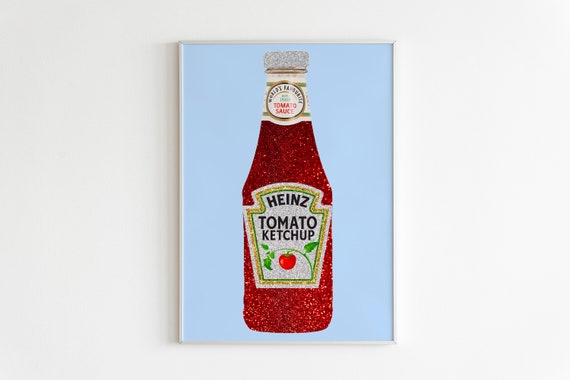The image showcases a framed piece of art displayed against a white wall. The art, centered within a metallic or white frame, is a vertical print featuring a light baby blue background. The primary focus of the piece is a depiction of a Heinz Tomato Ketchup bottle. This bottle is particularly eye-catching due to its glittery, red material reminiscent of the ruby slippers from The Wizard of Oz. The glitter extends to the label in the center, which reads "Heinz Tomato Ketchup" alongside an image of a tomato on a vine. The top label, stating "Tomato Sauce" and an indistinct word before it, appears more traditional, while the bottle's white lid is similarly bedazzled with glitter. The overall composition suggests a digital or photographic artwork that captures the vibrant and whimsical nature of the glittery ketchup bottle.